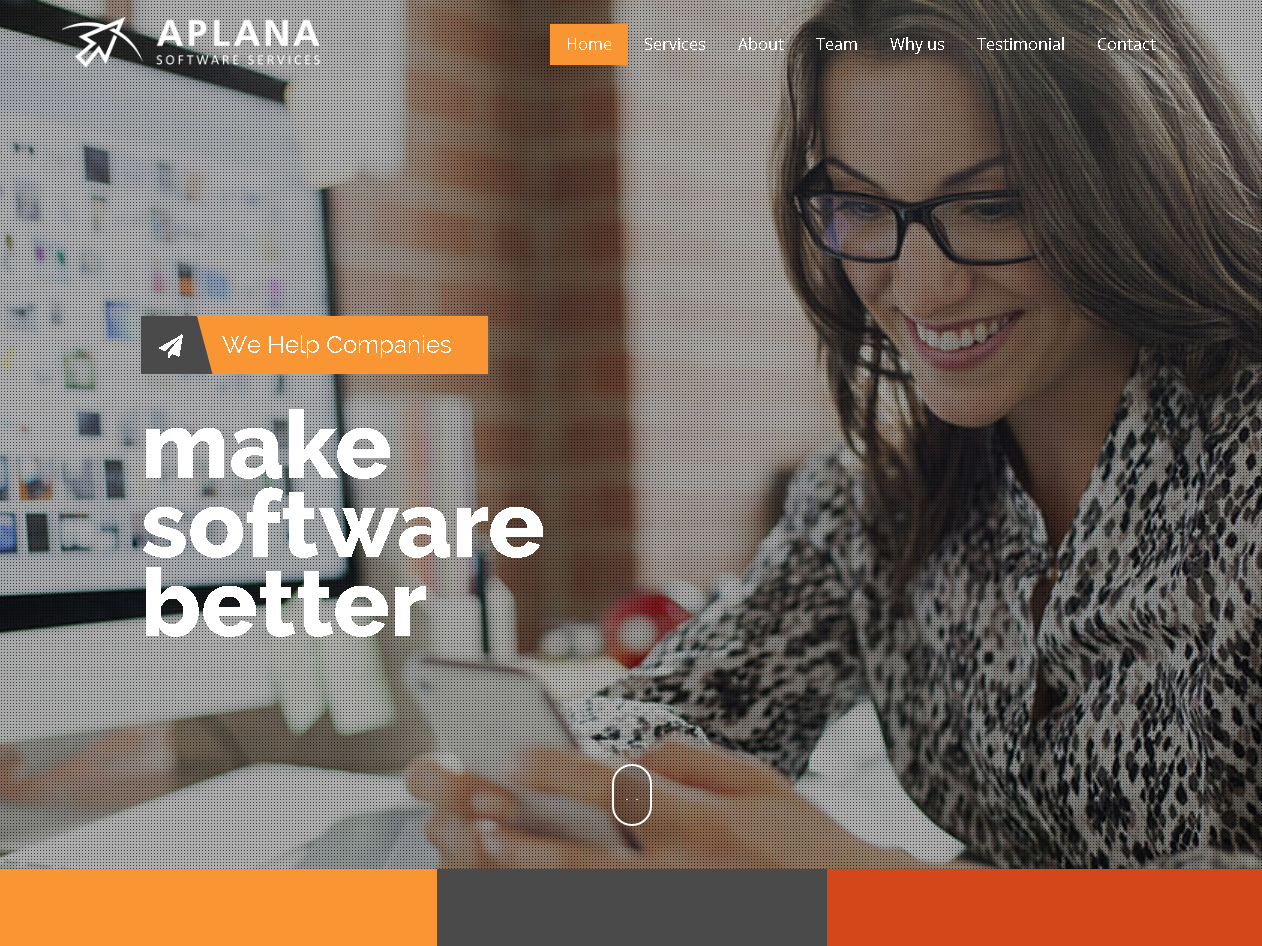This image, sourced from the App Planner website, prominently features the App Planner branding in the upper left-hand corner. The brand name "APP PLANNER" is displayed in bold, white uppercase letters immediately above the tagline "Software Services." Adjacent to the text is a distinctive logo resembling a mouse arrow pointing to the upper right, with a stylized, bendable line traversing the arrowhead.

The background image captures a woman engaged with a cell phone. Positioned predominantly on the right side of the frame, the woman appears to be in an office setting, seated at a desk. She has black hair and wears glasses, focusing intently on the device she holds with both hands, rested on the desk surface. On the left side of the image, a PC monitor is slightly visible, hinting at the workspace environment.

Overlaying the image and situated on the right side, the phrase "Make Software Better" is clearly presented in large, white font, spread across three lines, reinforcing the purpose and mission of App Planner.